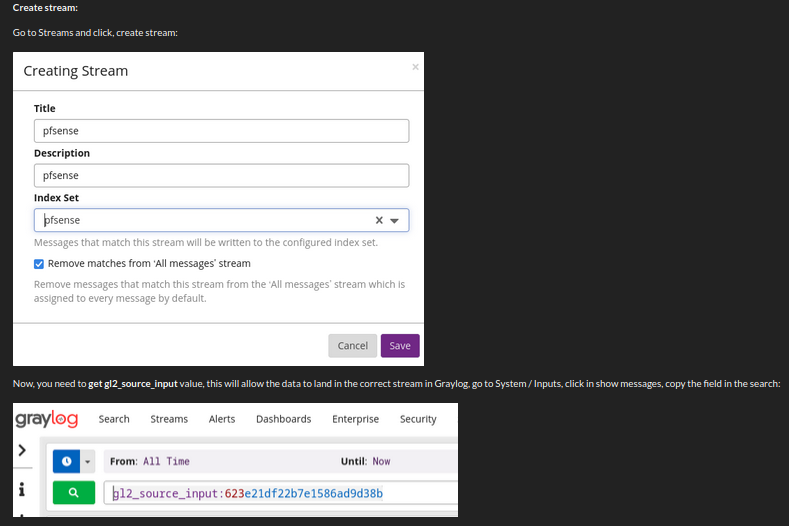The image displays a user interface from a website named Gray Log. In the top left-hand corner, there is prominently displayed text that reads "Create Stream." Directly below this instruction, additional guidance reads, "Go to Streams and click Create Stream."

A white, square window is central to the image. Inside this window, there are distinct fields for inputting a title, a description, and selecting an index set. In the bottom right-hand corner of this white window, there are two buttons: a light gray "Cancel" button and a purple "Save" button.

Below this area, in the bottom left-hand corner, there is a rectangular white window, which is also part of the Gray Log website interface, as indicated by the Gray Log logo in the top left-hand corner of the interface.

To the right side of the image, both the top right and bottom right corners are blank, featuring a black background color. This blank space extends across these areas.

Between the two aforementioned windows, at the center left of the image, there is a piece of white text that reads, "Now you need to get the source. This will allow the data to land in the correct stream in Gray Log. Go to System Inputs, click in Show Messages, copy the field in the search."